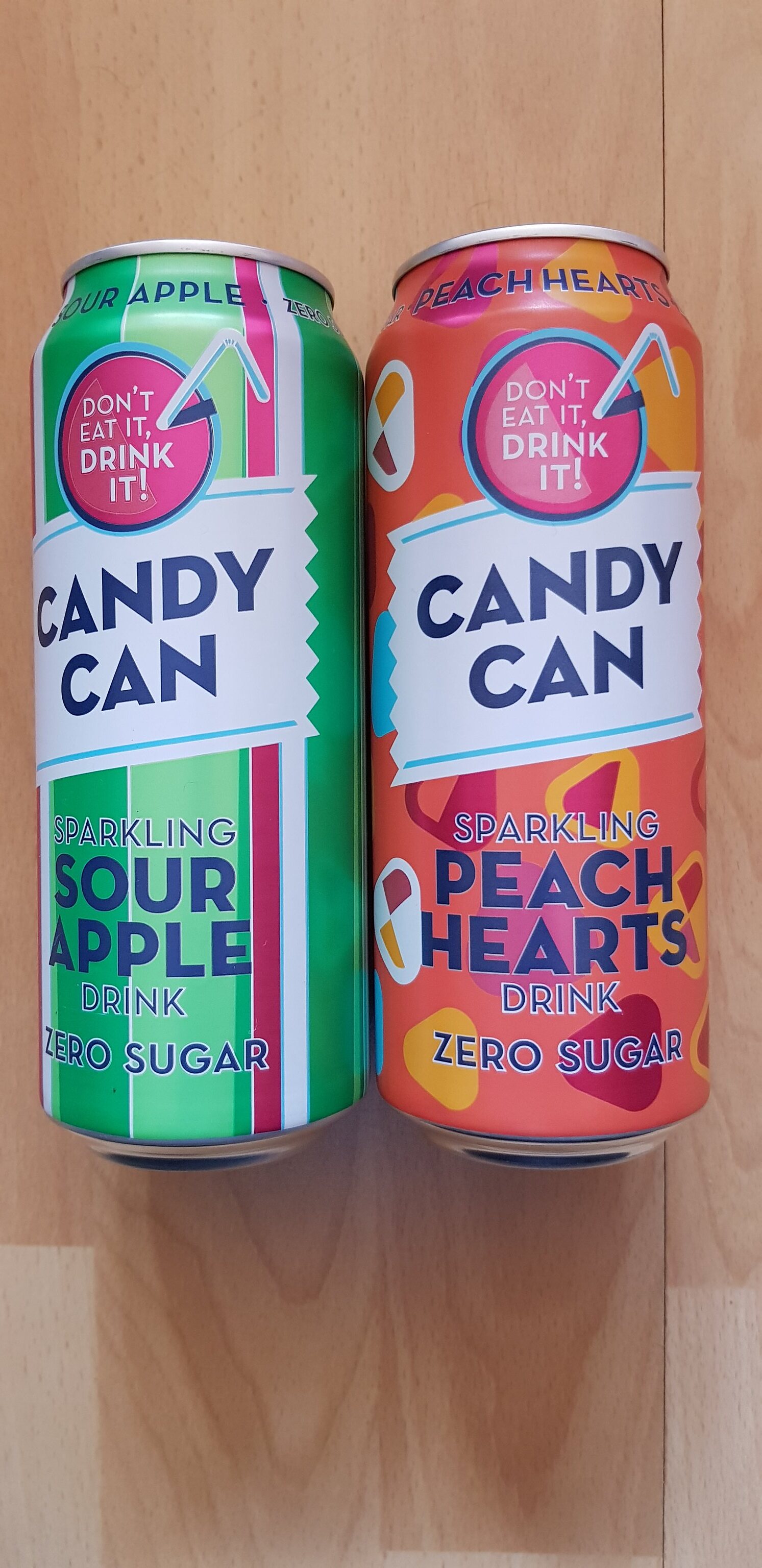In this vibrant image, we see two aesthetically-pleasing canned beverages from the brand Candy Can. The can on the left is an eye-catching green, while the can on the right boasts a lively blend of orange and pink hues, adorned with intricate designs. Each can features a distinctive pink circle above the brand name, Candy Can, illustrating a beverage with a straw, accompanied by the playful tagline, "Don't eat it, drink it." The flavors are prominently displayed at the top of each can, with the green can labeled as "Sour Apple" and the colorful can labeled as "Peach Hearts." Below, additional information clarifies that these are sparkling drinks with zero sugar, indicated by the text "Sparkling Sour Apple Drink, Zero Sugar" on the green can and "Sparkling Peach Hearts Drink, Zero Sugar" on the orange-pink can.